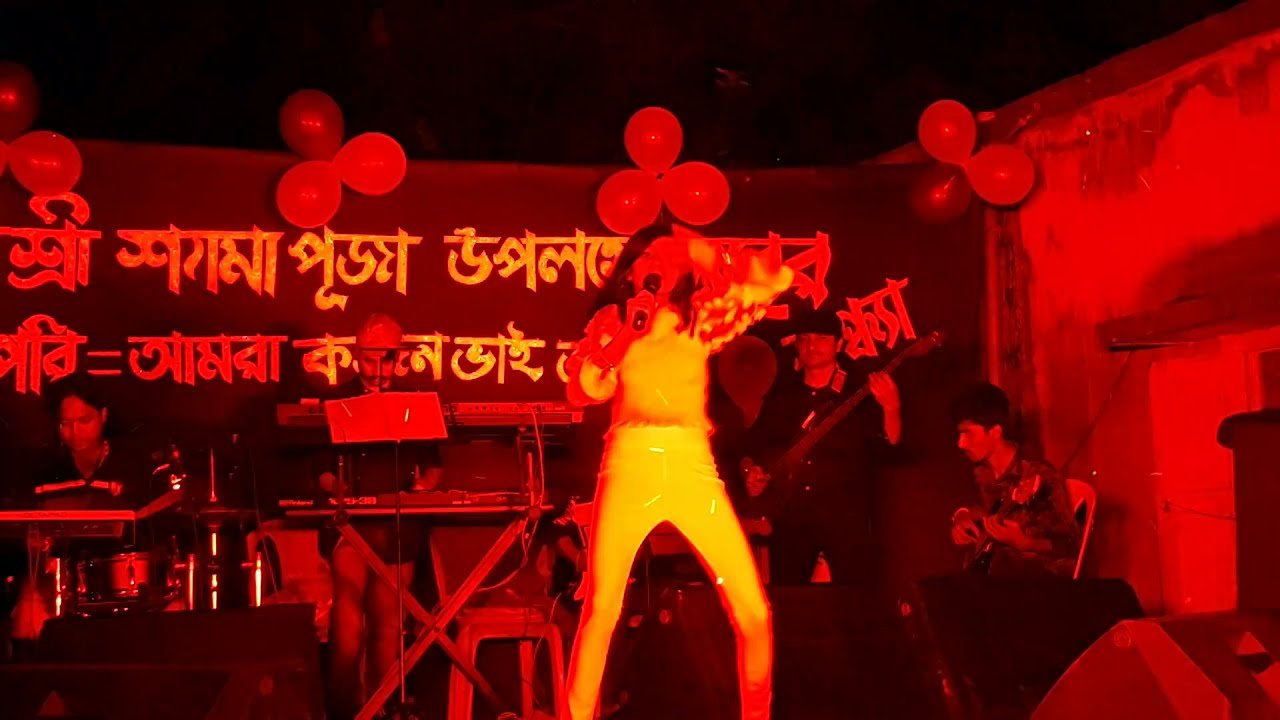In this photograph of a vibrant, red-tinted live concert, five band members take center stage, each playing different instruments. The scene is bathed in a bright red light, giving the entire setting a dramatic hue. At the forefront of the image stands the lead vocalist, a woman with long, dark brown hair, dressed in a white or yellow outfit that contrasts vividly with the red ambiance. She holds a microphone in her right hand while her left hand is extended towards the crowd, indicating her engaging performance.

To her right, there is a dark-haired man sitting in a chair, skillfully playing an electric guitar. Next to him stands another man, donned entirely in black with a black baseball cap, who is passionately playing a bass guitar. On the opposite side of the vocalist, to her left, a bald man with a black mustache stands behind a two-level keyboard, deeply engrossed in his music. Further left, near the edge of the image, another dark-haired man, distinguishable by a black shirt with a white stripe, is seated behind a drum set, adding rhythmic beats to the performance.

The backdrop features a black wall adorned with clusters of balloons pinned in groups of three, creating a festive air. Silver foreign text, possibly in Hindi or Arabic, is seen beneath the balloons, adding an exotic touch to the setting. Overall, the photograph captures the dynamic energy and immersive atmosphere of a live band performance, frozen in a moment of musical fervor.